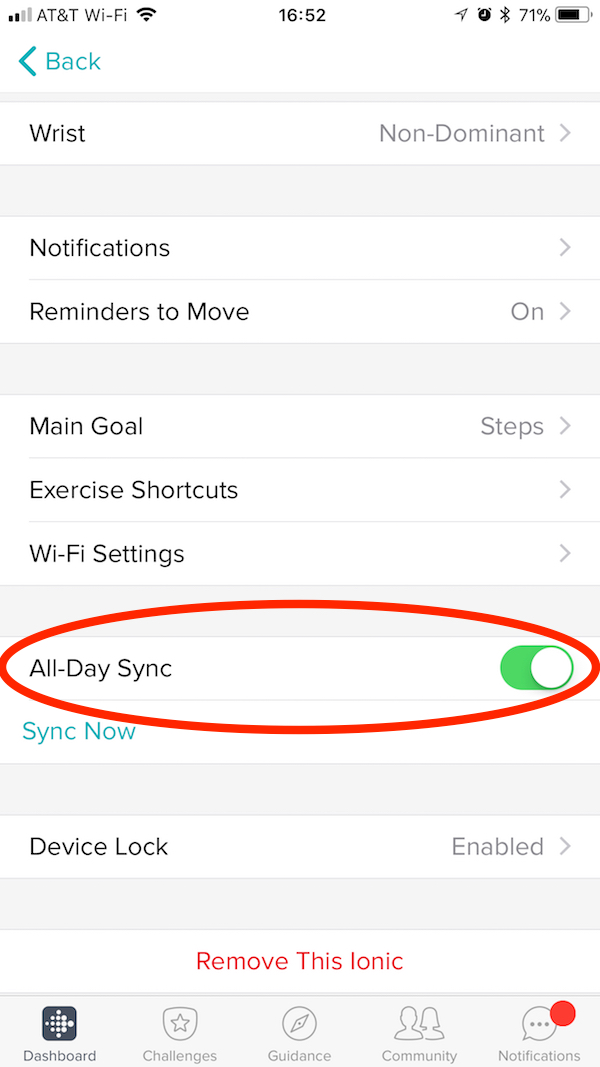This is a detailed and organized description of the screenshot:

---

The screenshot captures the settings menu of a fitness tracking app on an iPhone. The status bar at the top displays several indicators: the time, set to 16:52 in a 24-hour format; a Wi-Fi connection; the data signal strength at approximately 25%; a battery level at 71%; GPS connectivity, denoted by an arrow icon; an alarm icon indicating an alarm is set; and an active Bluetooth connection.

Below the status bar, at the top left corner, there is a blue arrow labeled "Back," serving as a navigation element for the user to return to the previous screen. The settings options are presented in a descending list. The first option shows "Wrist" with "Non-dominant" currently selected. Following this, there is a section for "Notifications," and the "Reminders to Move" feature is turned on. The "Main Goal" is set to track steps, although this can be adjusted by the user. At the bottom are "Exercise Shortcuts" and "Wi-Fi Settings," which appear to lead to their respective submenus.